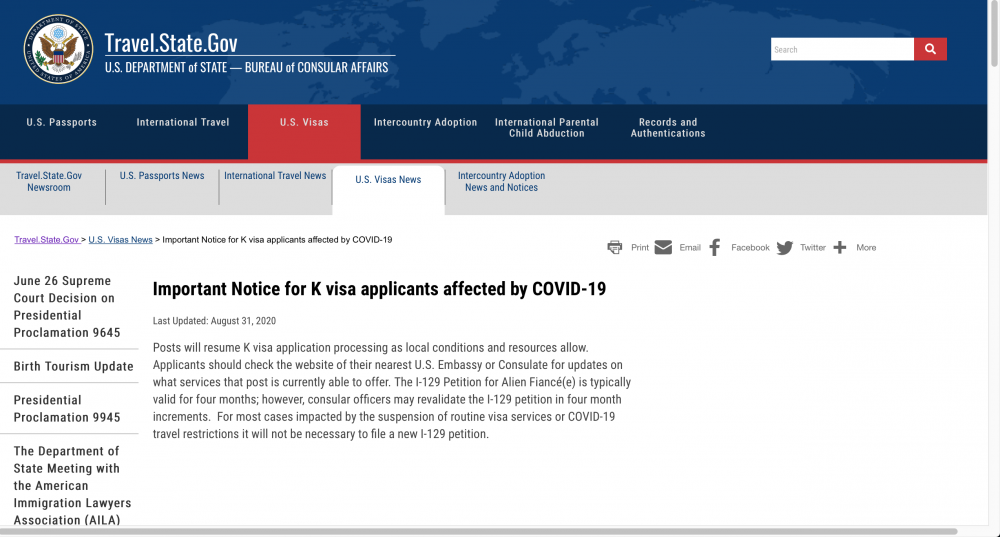This image showcases the homepage of the travel.state.gov website, managed by the U.S. Department of State's Bureau of Consular Affairs. In the top left corner, the official logo is prominently displayed, featuring the emblem of the Department of State, United States of America, along with the site URL and Bureau of Consular Affairs designation. 

Navigational links are neatly listed, providing access to essential categories such as U.S. Passports, International Travel, U.S. Visas, Inter-country Adoption, and International Parental Child Abduction. Additionally, a category for Passports and Authentications is available.

A search field is positioned in the top right corner of the page, enabling users to conduct specific queries. Below the navigation links, notable text alerts visitors to important announcements, including an important notice for K visa applicants affected by COVID-19 and information about the Supreme Court decision on Presidential Proclamation 9645 dated June 26th. This detailed layout ensures that users can easily find pertinent information related to consular services and travel advisories.